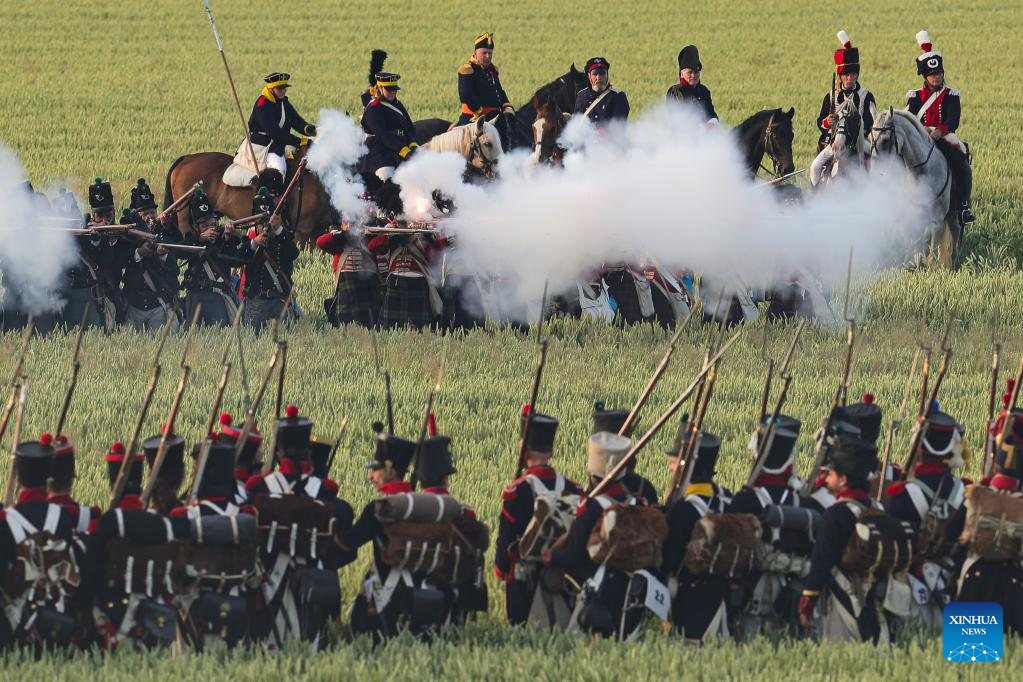In this detailed color photograph of a war reenactment, we see an intense battle scene set in a tall grass field, with grass reaching up to the soldiers' hips. The image captures two rows of infantrymen from a European army, likely from the Napoleonic era, indicating French and British troops. The soldiers in the foreground, wearing dark blue uniforms with red collars or shoulders and tall black hats—some adorned with red pom-poms—are facing away from the photographer. These men hold rifles with bayonets and carry brown leather or animal skin backpacks.

About 12 to 15 feet ahead, another line of soldiers faces towards the photographer. They wear a mix of blue blazers with red stripes, tartans suggesting Scottish units, and gray pants. Thick clouds of musket smoke obscure their faces, highlighting the intensity of the confrontation. At the distant part of the field, commanders or officers on horseback are visible behind the line of kneeling and firing troops. The background figures are clad in red and black uniforms, intensifying the scene with their readiness for battle.

The center of the image is dominated by white smoke from the firing muskets, adding a dynamic element to the visual. Notably, a blue label in the bottom right corner of the photograph reads "XINHUANEWS" in white lettering, providing a hint about the source or publication of this vivid depiction of historical reenactment.